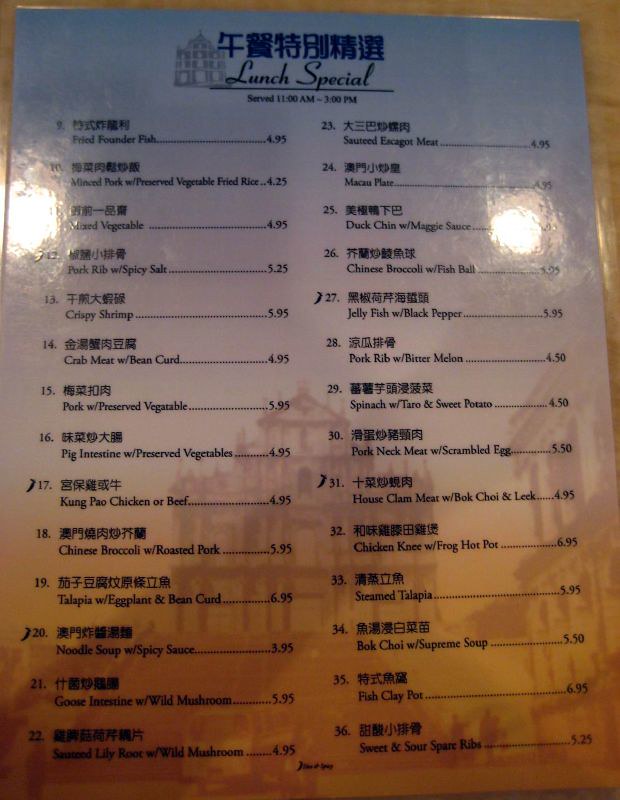This photograph captures a laminated lunch special menu at a Chinese restaurant. Dominating the visual is the elegant header "Lunch Special" written in cursive, accompanied by traditional Chinese characters above it. Adjacent to the header on the left, a traditional Chinese building logo adds a touch of cultural authenticity.

The menu is organized into two vertical columns, each superimposed over a faded background image of a classical Chinese building, enhancing the traditional ambiance. Each lunch special is meticulously numbered, with the dish name presented first in Chinese characters, followed by its English translation below. 

Highlighted menu items include "House Clam," "Spinach with Taro," "Pork with Preserved Vegetable," and "Crab Meat with Bean Curd." The corresponding prices are listed to the right, ensuring clarity and ease of selection for diners. The detailed and organized layout reflects a harmonious blend of cultural elements and practical design, inviting guests to explore the diverse lunch offerings.